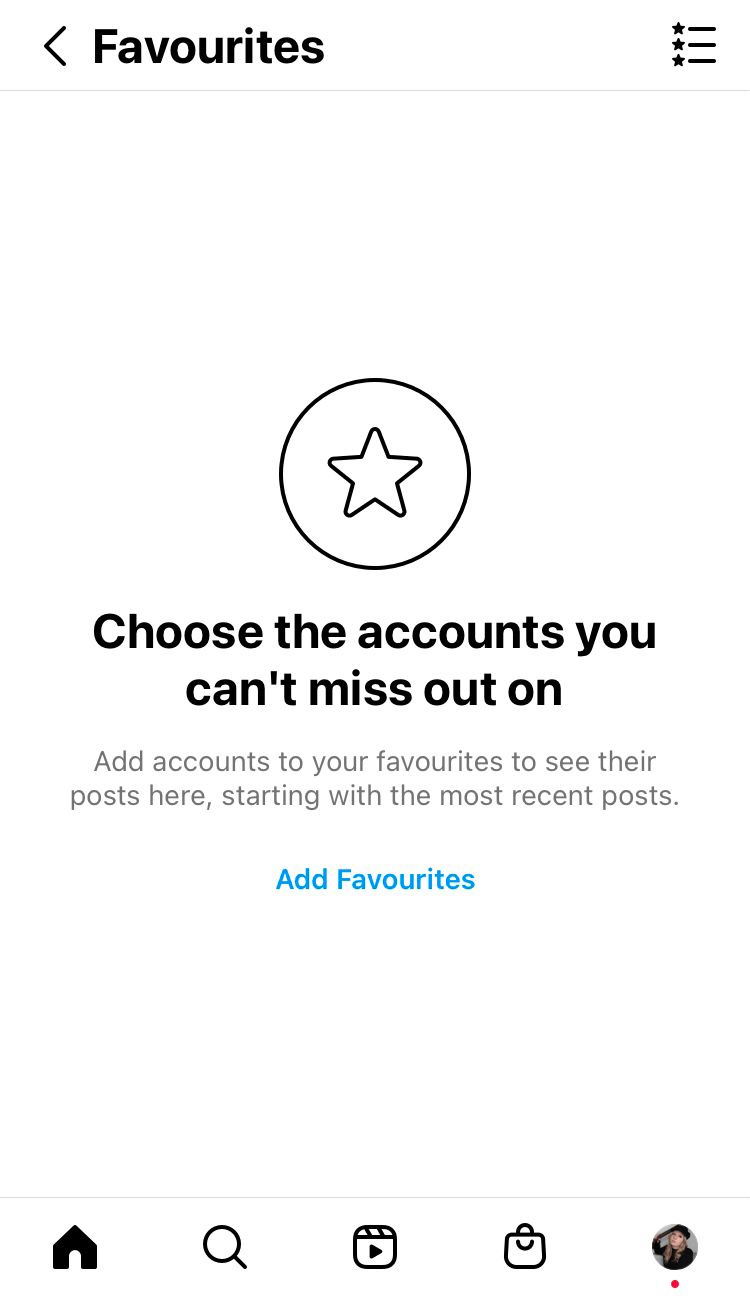The image appears to be a screenshot of a mobile app interface, likely from social media applications common on iPhone and Android devices.

At the very top of the image, there's a black, sideways V-shaped icon pointing left. To its right, bold black letters spell out "Favourites" with the British spelling. Adjacent to this text, a small symbol with three star bullet points and three black lines lies next to it on the right. A faint gray line runs beneath these elements.

The background of the image is predominantly white. In the center, there’s a black circle containing a white star with a black outline. Below this circle, bold black text states: "Choose the accounts you can't miss out on." Underneath, additional gray text reads: "Add accounts to your favourites to see their posts here, starting with the most recent posts."

An aqua blue link labeled "Add Favourites" with the British spelling appears below the descriptive text. Further down, another very faint gray line runs across the screen. 

At the bottom of the image lies a navigation bar with various icons, arranged from left to right: a black house icon, a black magnifying glass, a black square with a play button, a black shopping bag, and on the far right, an avatar icon of a person, likely wearing a black outfit. The avatar has a small red dot beneath it, hinting at a notification.